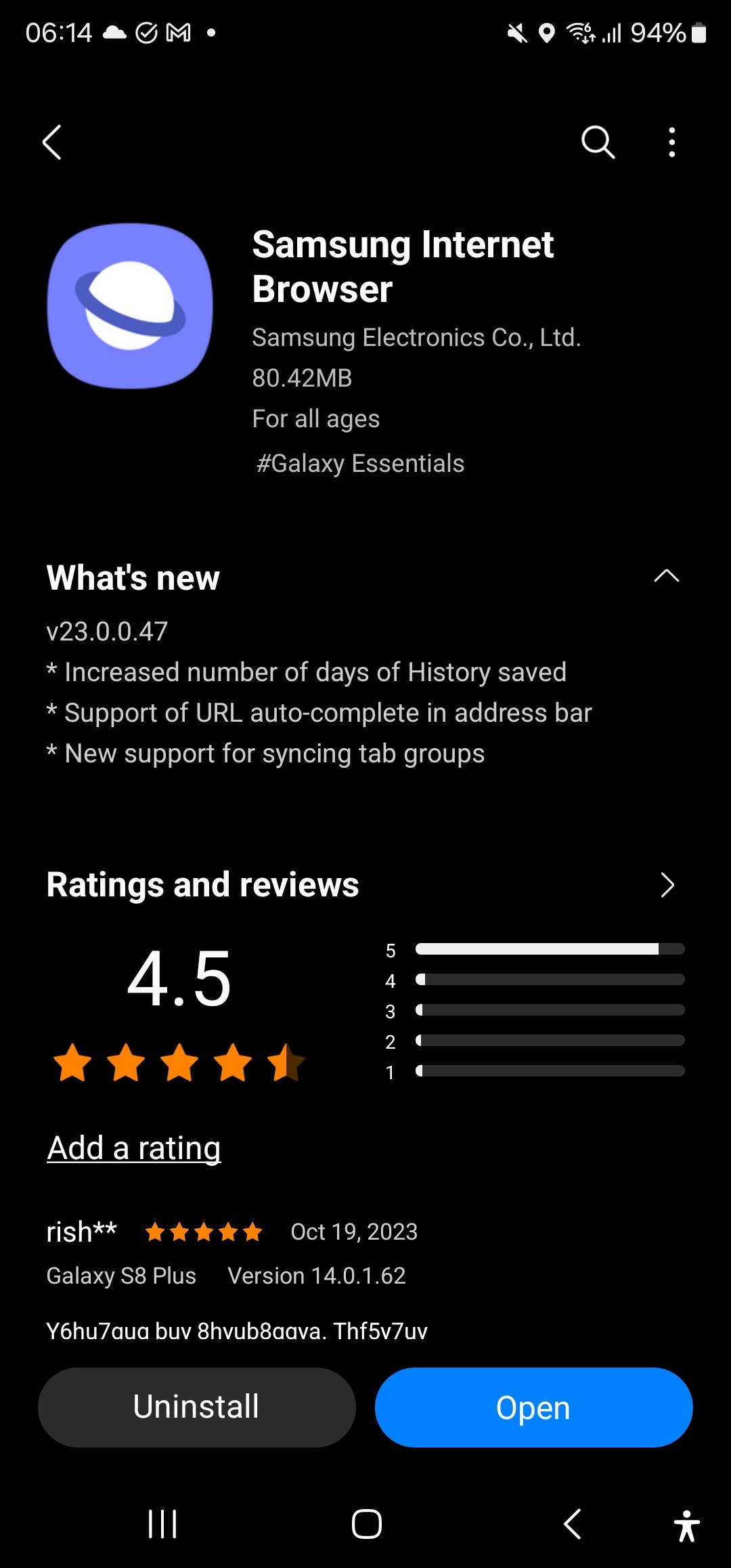This vertical mobile screenshot showcases a detailed view of the Samsung Internet Browser page within the app store. At the top, the status bar displays the current time, along with various icons on the left, and the battery percentage (94%) accompanied by more icons on the right. The navigation bar beneath features a left arrow button, a search button, and a vertical ellipsis, all set against a black background.

Dominating the upper section of the page is the Samsung Internet Browser logo, which depicts a planet set within a light blue circular background. Adjacent to the logo, "Samsung Internet Browser" is displayed in bold white text. Below this title is the "What's New" section, highlighted by an upward scroll button on the right. This area provides details about recent updates to the browser.

Further down, the "Ratings and Reviews" section boasts an overall rating of 4.5 stars, visually represented by four and a half orange stars. To the right, a slider bar ranks user ratings from five to one, with the number five showing a nearly full white line. Beneath the rating visuals is a prompt to "Add a Rating."

A recent review by a user named RISH****, who rated the browser five stars on October 19th, 2023, is also visible. Concluding this comprehensive page are two prominent buttons: a grey "Uninstall" button and a blue "Open" button for quick access. At the very bottom, the footer displays four essential icons.